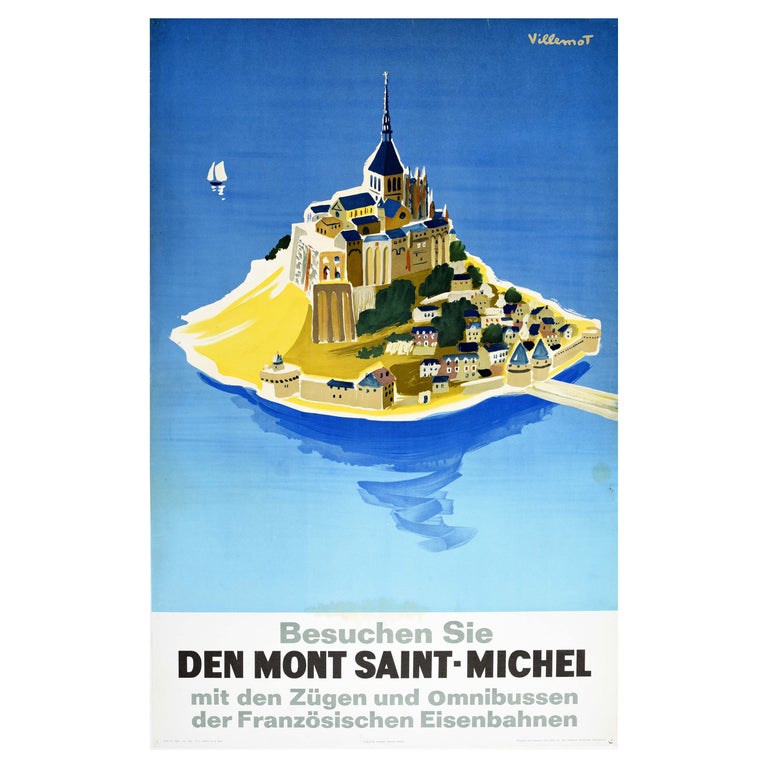The poster is an animated, possibly computer-generated, depiction of Mont-Saint-Michel, set against a gradient blue background representing the water, transitioning from light blue at the bottom to darker blue towards the top. Dominating the scene, Mont-Saint-Michel stands on a small island with yellowish-whitish land. The central feature is a castle with a dark roof and a prominent blue spire, situated atop a hill. Surrounding the castle, a protective wall encloses village buildings in various shades of yellow, brown, and tan, with some roofs featuring blue tips. The village spreads down the hill, leading to a drawbridge crossing over the water. At the bottom of the poster, there's a white rectangle containing text in a dark gray, foreign language, which reads "Buchen Sie den Mont-Saint-Michel mit den Zugen und Omnibussen der französischen Eisenbahnen." In the top right corner, the names "Villamat" and "Scripp" appear in gray cursive script.